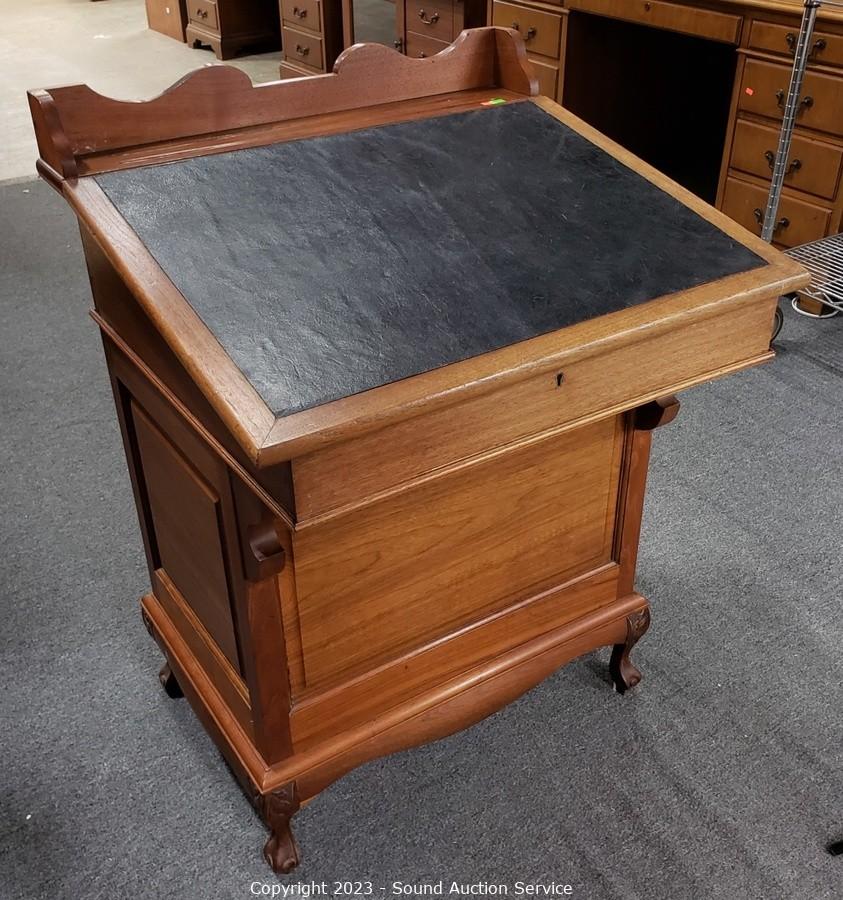The image captures an antique writing desk or lectern, typical of the late 1800s to early 1900s. Crafted from cherry wood or a similar brown wood, it stands slim and short with a distinguished, geometrical design. The top features a black slate chalkboard writing surface and a decorative wavy pattern. A keyhole is positioned in the front, indicating a possible lift-up mechanism for storage within. Below the desk, it sits on a black tarp, adding contrast to the scene. In the background, there are matching larger wooden desks, their cherry wood hue resonating with the main piece. These desks are partially visible, showing the drawers and the under-desk cavities meant for chair placement. The floor is adorned with a gray carpet, enhancing the showcase environment. Additionally, a corner of a metal cart used for larger items is slightly visible, suggesting the setting is a furniture shop or thrift store. At the bottom of the image, white text reads "Copyright 2023 Sound Auction Service."